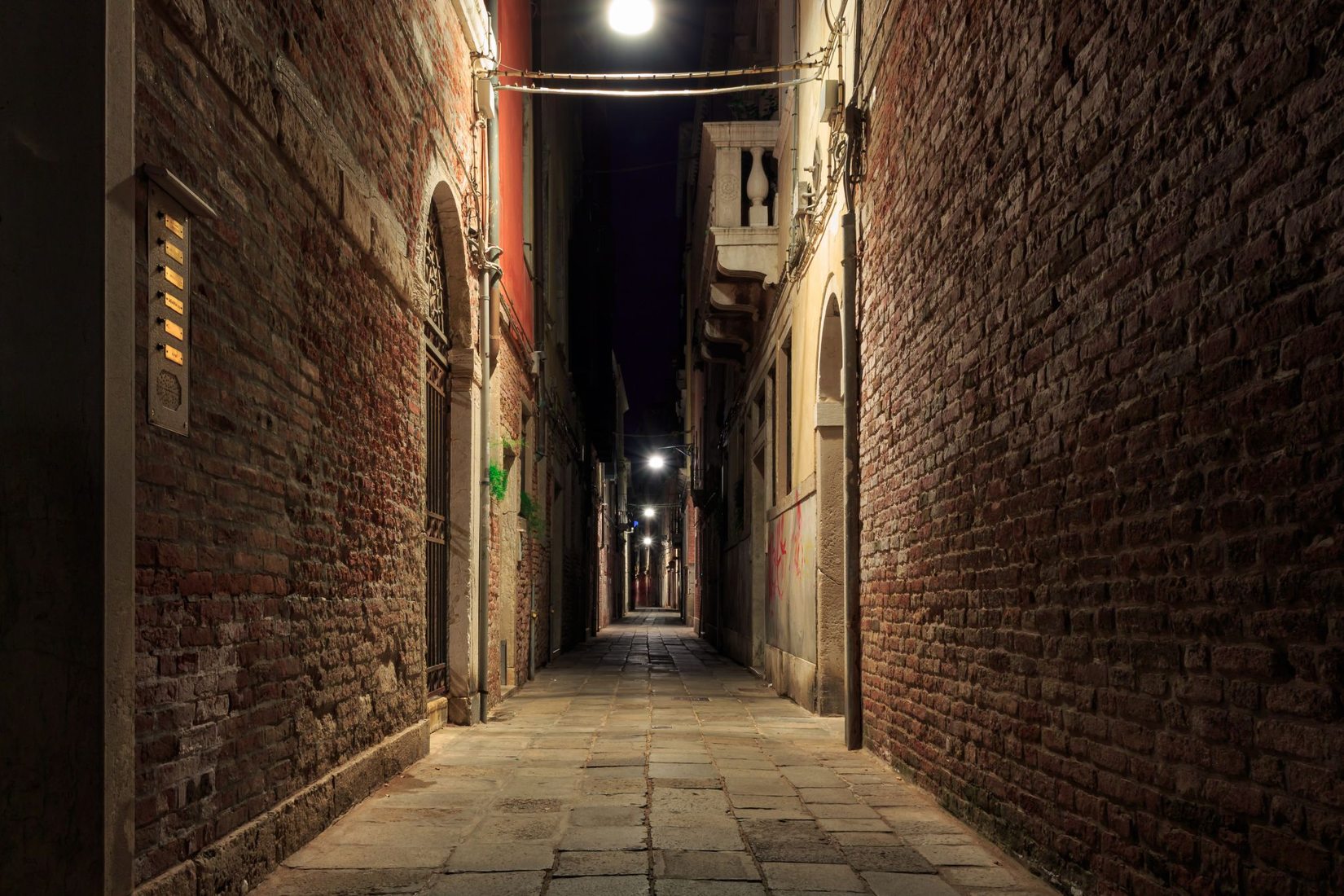This well-lit alleyway is framed by tall, red brick buildings on both sides, which rise to at least two or three stories. The path itself consists of square cobblestones in varying shades of light and dark brown. Along the left wall, there's a rectangular plaque with gold names printed on it near a door equipped with a series of six contact buttons. From the top of both walls hang ropes, adding an intricate detail to the scene. Further down the alley, an arched entrance is visible, leading into the building. In the background, a white balcony is seen emerging on the right side. Numerous street lamps illuminate the alleyway, casting their light on the cobblestone path. The sky above is dark, with the moon prominently visible, adding a natural source of illumination. Strings of lights hang across the alley, further brightening the scene, and contributing to the overall sense of a dimly lit yet navigable urban passageway.